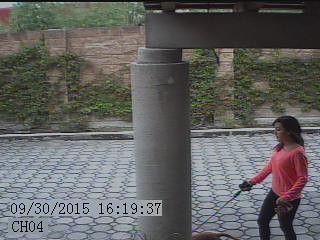A small horizontal rectangular image from a home security camera, dated 09/30/2015 at 16:19:37, shows a woman wearing a pink top and black pants walking an animal on a leash, likely a dog. The scene is set on a tiled patio or courtyard with circular, multi-shaded tiles in hues of gray and light purple. Central to the image is a large gray concrete column supporting a platform, with a distant background featuring a stone wall adorned with green ivy. The time, date, and camera channel (CH04) are displayed in the lower left corner, capturing this moment in a somewhat dark setting with subtle illumination.